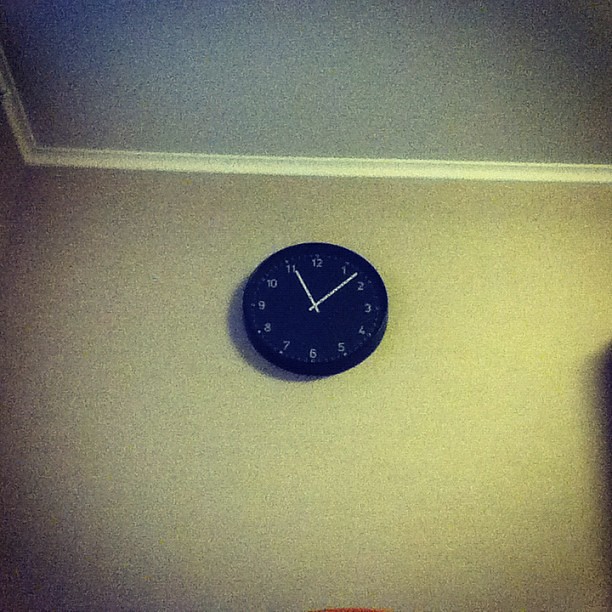The image depicts an interior wall characterized by a unique color scheme and texture. The top portion of the wall is painted gray, followed by a prominent white strip running horizontally across its midsection, and the bottom part is beige. A small part of a cabinet is visible in the corner. Centrally mounted on the wall is a thick, black plastic clock with a black face. The clock features standard white numerals and slim, white plastic hands. Both the wall and ceiling exhibit a noticeable textured finish, giving them a bumpy appearance rather than a smooth surface.